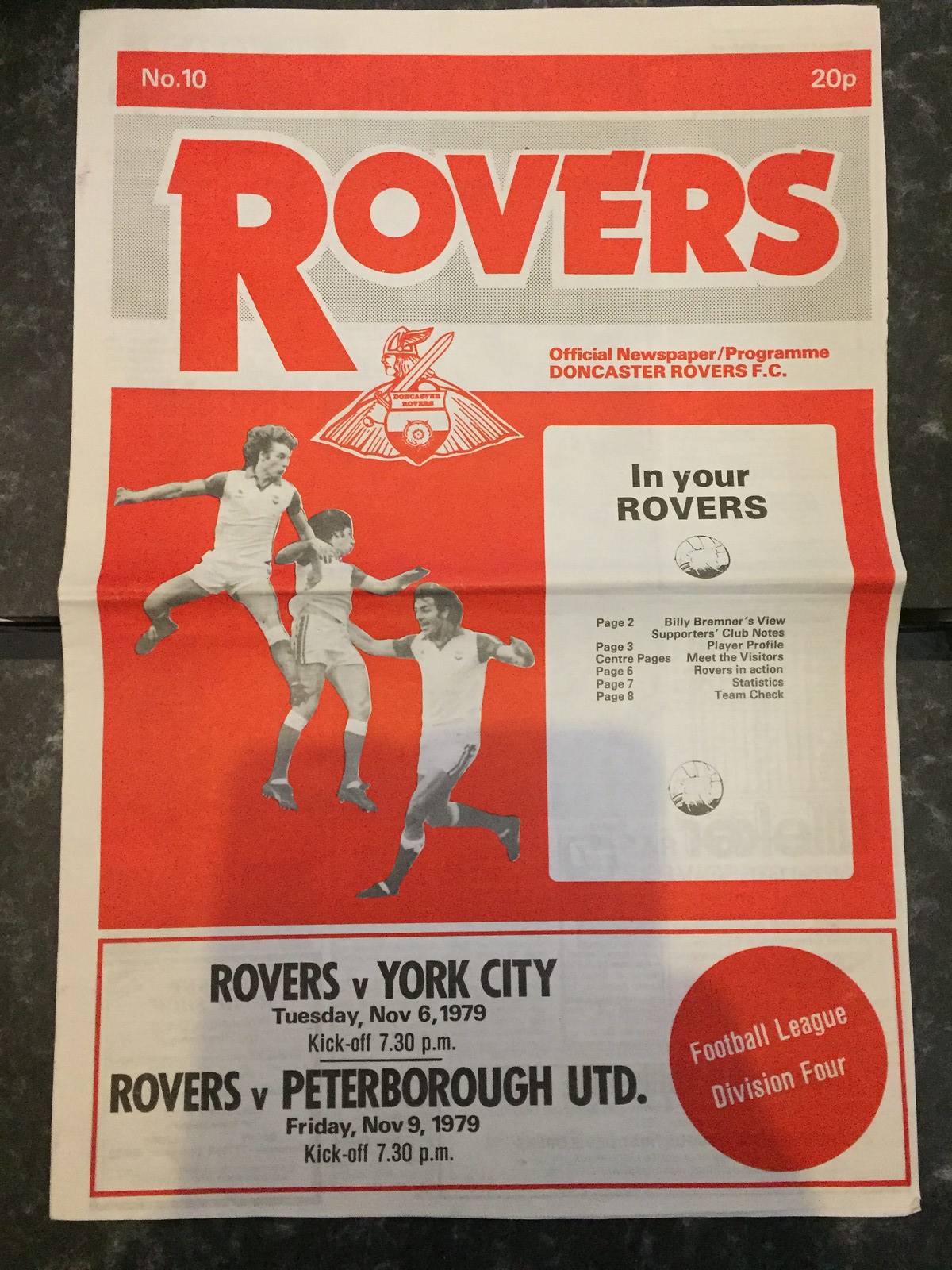This is a detailed photograph of an old newspaper or sports program from England, specifically for the Doncaster Rovers Football Club. The image shows a rectangular, red, gray, and white program. At the top, a red banner displays the issue number "10" on the left and the price "20p" on the right. Just beneath it, a large gray banner with red lettering trimmed in white reads "Rovers". Below this banner, against a white background, the text reads "Official Newspaper/Program Doncaster Rovers F.C.".

Centrally located is the symbol of the Rovers alongside three black-and-white photographs of players in different action poses, set against a red background. These players are all depicted wearing white jerseys and shorts with dark socks. To the right of these images is a black text box labeled "In Your Rovers", accompanied by a drawing of a soccer ball and additional small text beneath it.

The bottom section of the program features upcoming match details outlined in a red triangular box: "Rovers v. York City Tuesday November 6 1979 kickoff 7.30 p.m." and "Rovers v. Peterborough UTD Friday November 9 1979 kickoff 7.30 p.m." On the right side of this section, a red circle contains the text "Football League Division IV" in white letters. The entire composition captures a detailed snapshot of the historical sports publication, reflecting the club's identity and upcoming fixtures.